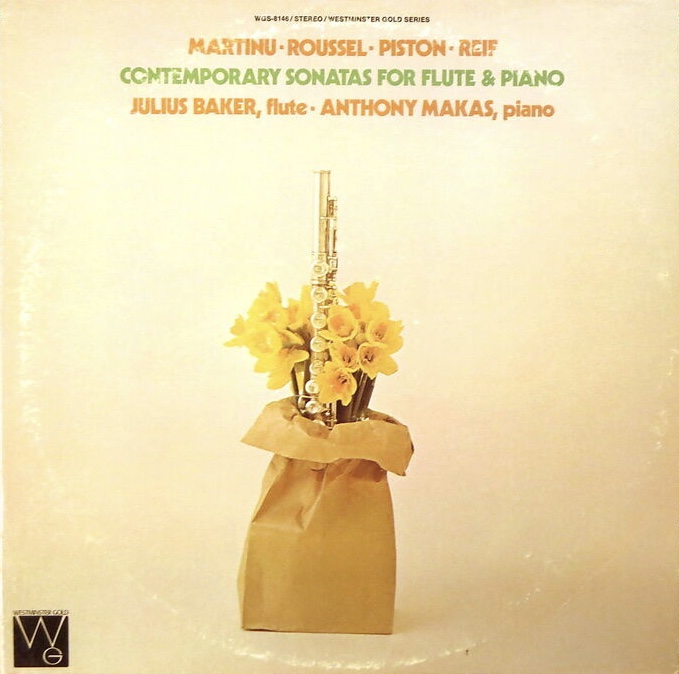This is an off-white poster featuring a photograph of a brown paper or cardboard bag filled with yellow flowers, each with long green stems, and a metallic flute that appears pale brown or golden in color. The flute is positioned upright in the middle of the flowers. At the top of the poster, written in orange text, are the names "Martinu, Roussel, Piston, Reef," followed by the title "Contemporary Sonatas for Flute and Piano." Below this, in green text, it states the performers: "Julius Baker, Flute, Anthony Marcas, Piano." Additional orange text is located at the top, middle, and lower sections of the image. In the bottom left corner is a black square containing the white letters "WG." The background has soft pink and orange tones, enhancing the overall musical theme of the poster.